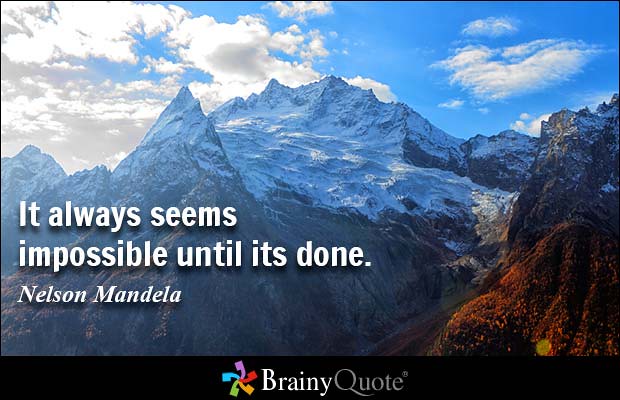The image captures a breathtaking mountain range with snow-capped peaks and a few areas of exposed rock, creating a striking portrayal of natural beauty. The mountains dominate the central two-thirds of the frame, giving a grand sense of scale, while the sky above features a mix of vibrant blue and fluffy white clouds scattered throughout. Towards the left bottom part of the image, a motivational quote in white text reads, "It always seems impossible until it's done. - Nelson Mandela." Below this, a black banner runs horizontally across the bottom, featuring a colorful flower-like rainbow symbol in shades of blue, purple, red, orange, yellow, and green next to the text "Brainy Quote." The composition, enriched by its vivid colors and inspiring message, resembles a postcard or a social media graphic designed to uplift and motivate.